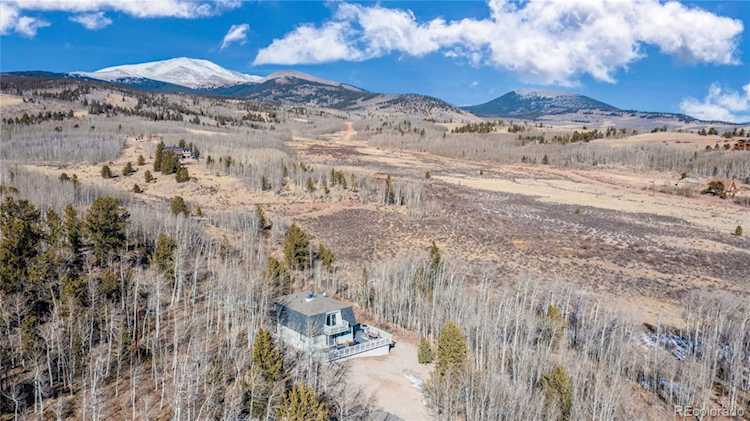In the center of this wilderness landscape, a unique house stands with no neighbors or roads in sight. The house has a square shape, and its lower portion features a large deck with a railing. The upper level is gray while the lower level is white, and it has a large window with a small balcony attached. Surrounding the house is a mix of trees, most of which have lost their leaves, indicating fall or winter, with scattered pine trees that still retain their green needles. The ground is mostly brown, suggesting that much of the plant life has died off. In the vast background, there's a panoramic view of hills and mountains, with one mountain appearing snow-capped. The blue sky with hovering clouds completes this remote, tranquil setting, which appears to stretch on for miles.